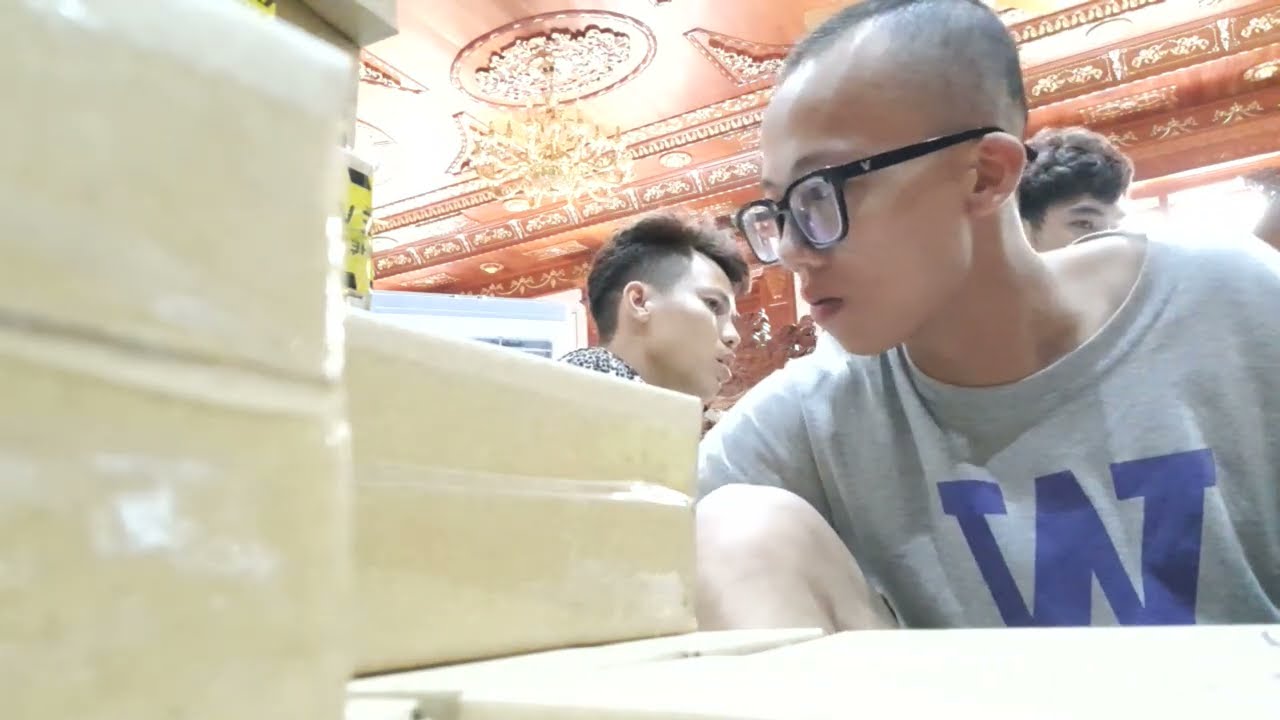This indoor photograph captures a richly decorated setting featuring a high ceiling adorned with reddish-orange hues and intricate molding. At the center of the ceiling, a decorative plate supports a gold chandelier. In the foreground, a young person with a buzz cut and thick, dark-framed glasses sits with knees pulled up to the chest, looking off to the right. This individual wears a gray t-shirt emblazoned with a dark blue "W". To his left and slightly behind, a glimpse of another person’s face and hair is visible. Over his right shoulder, another short-haired individual gazes inquisitively towards the right. The room is vibrant, with brown walls carrying various elaborate designs, enhancing the luxurious ambiance. In front of the seated individual, there is a table with some brown cardboard boxes on it, adding another layer to the scene's detailed composition.